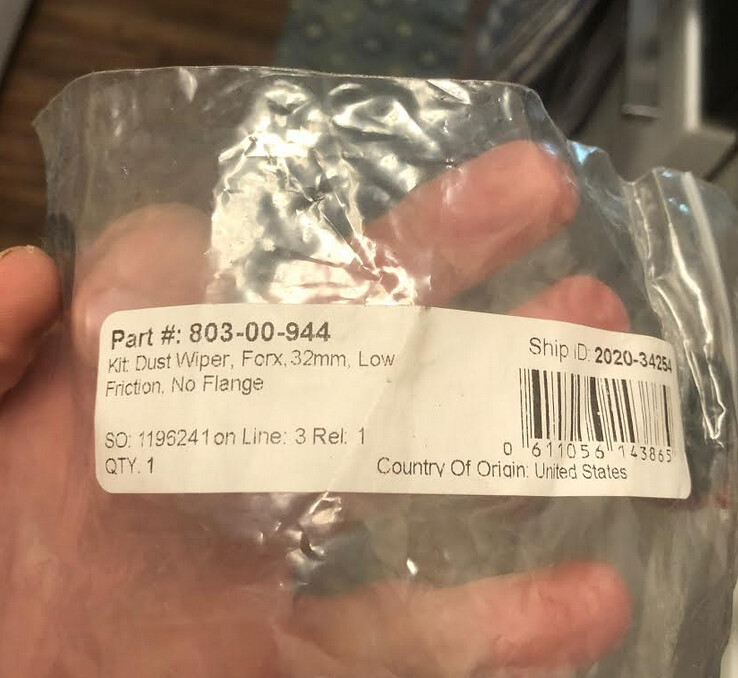A close-up photograph features a hand holding a translucent plastic bag in a kitchen setting. The focal point of the image is a white label affixed to the front of the bag. The label, densely packed with text, reads: "Part Number 80300944, Kit Dust Wiper, Forks, 32mm, Low Friction, No Flange. SO1196241 on line 3, RHEL 1, Quantity: 1, Ship ID: 2020 3454". Additionally, a barcode labeled "Country of Origin: United States" is visible. In the background, the scene is set in a kitchen, characterized by a warm wood floor, a kitchen mat, and an oven, providing context to the domestic environment where the image was captured.